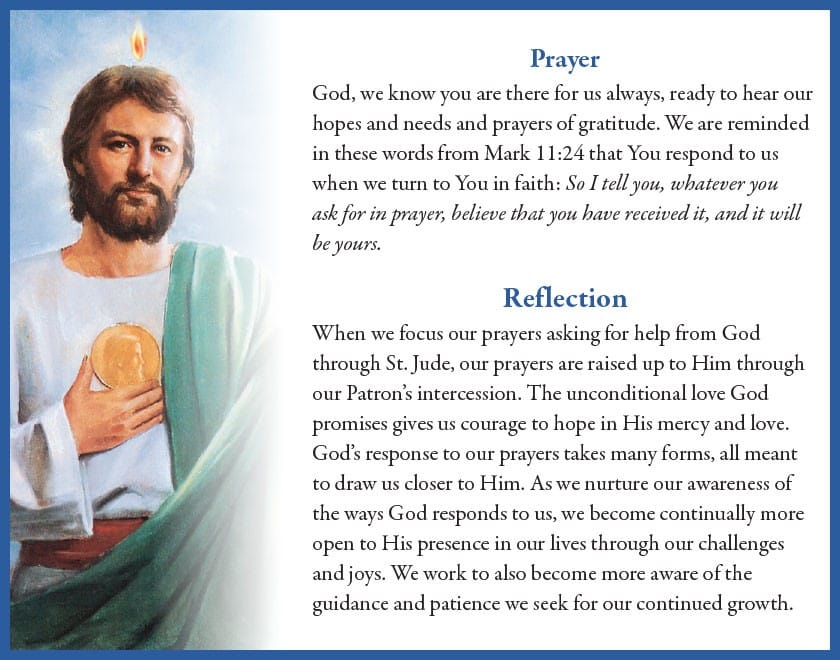This color illustration, possibly a prayer card, features a detailed drawing of a Caucasian man, resembling Jesus, on the left side. He has brown hair, a full beard, and is adorned in a white tunic with a green robe draped over his shoulder and a red belt around his waist. He holds an ornate gold medallion over his chest. Behind him is a light blue background, with an orange flame-like symbol above his head that adds a spiritual nuance. The right side of the image contains two paragraphs of text against a white backdrop. The top paragraph, titled "Prayer" in blue text, reminds us of God's readiness to hear our hopes and needs, referencing Mark 11:24: "Whatever you ask for in prayer, believe that you have received it, and it will be yours." Below that, a section titled "Reflection" in blue text discusses the power of prayers through St. Jude, emphasizing God's unconditional love and the many forms of His response. The entire image is encapsulated in a blue square border.